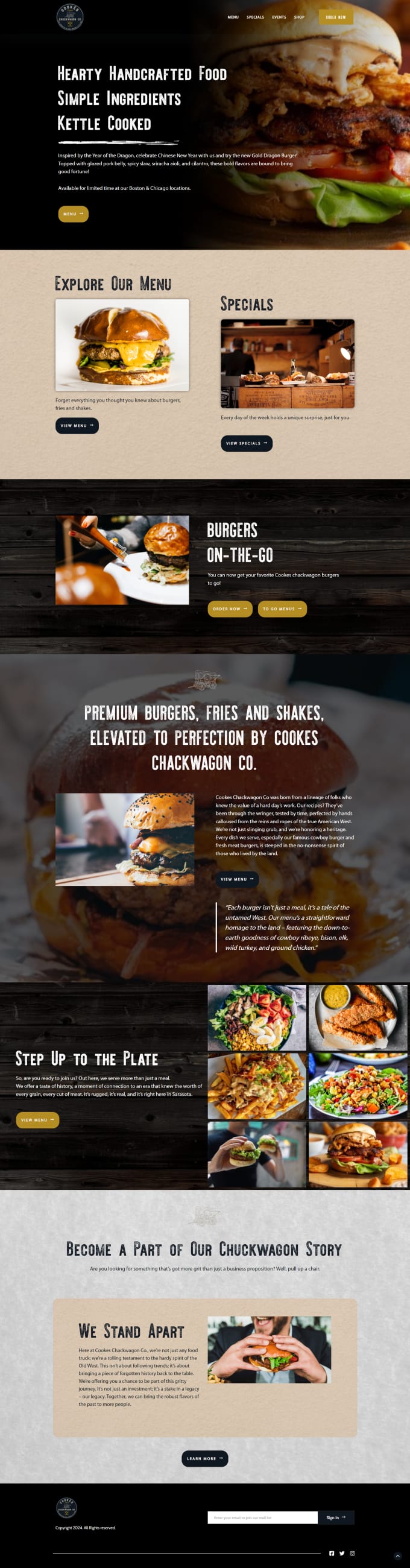Caption:
"The image depicts a cozy dining environment at a burger restaurant known for its hearty, handcrafted food made from simple ingredients and kettle-cooked methods. The top section of the image features a black background with a partially obscured, horizontally-stretched logo. On the right, there is a detailed view of a mouth-watering hamburger showcasing all its components. On the left side, the phrases ‘hearty, handcrafted food,’ ‘simple ingredients,’ and ‘kettle cooked’ are prominently displayed. Below this text, there is an orange button with unreadable white text.

Navigational options are located at the top-right edge, above the hamburger, including 'Menu,' 'Specials,' 'Events,' 'Shop,' and another unreadable orange button. The next section has a tan background with two photos: one of a hamburger with the caption ‘Explore our menu’ and another labeled ‘Specials,’ each accompanied by a black button beneath it.

Further down, there is a background photo of a hamburger on a white plate with the title ‘Burgers on the go.’ The text below reads, 'You can now get your favorite Cook’s Hamburger or Chuck Wagon burgers to go. Order now,' followed by two yellow buttons labeled ‘Order Now’ and ‘To Go Menus.’ The entire scene celebrates the indulgence of classic fast-food favorites like hamburgers, fries, and shakes, elevated to perfection by Cook’s Chuck Wagon Co."